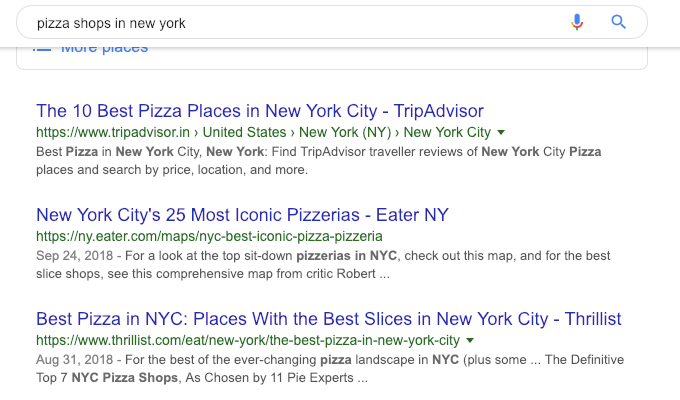The screenshot showcases a Google search results page with the query "pizza shops in New York" entered into the search bar, which also features a microphone icon and a magnifying glass icon on the right. The search yields three significant results:

1. **Best 10 Pizza Places in New York City - TripAdvisor**  
   *URL:* from.tripadvisor.in  
   *Snippet:* "Best pizza in New York City, New York: Find TripAdvisor travel reviews of New York City pizza places and search by price, location, and more."

2. **New York City's 25 Iconic Pizzerias - Eatery NY**  
   *URL:* nyeatery.com (displayed in green)  
   *Snippet:* "September 24, 2018. For a look at the top sit-down pizzerias in New York City, check out this map, and for the best slice shops, see this comprehensive map of Critic Robert..."

3. **Best Pizza in New York City: Places with the Best Slices - Thrillist**  
   *URL:* thrillist.com/eat/new-york (displayed in green)  
   *Snippet:* "August 31, 2018. For the best of the ever-changing pizza landscape in New York City..."

Each search result provides a URL and a brief description of what can be found on the respective pages, emphasizing reviews, locations, and recommendations for both sit-down pizzerias and slice shops in New York City.